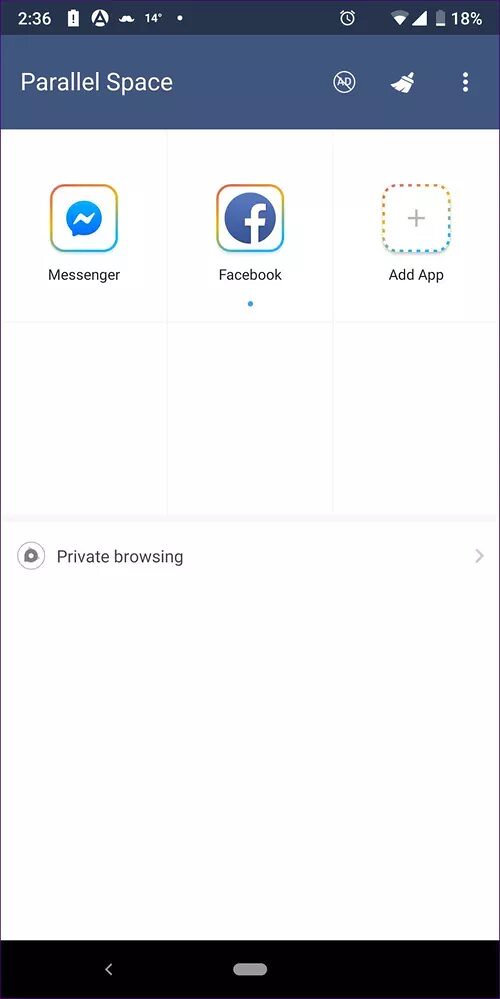This screenshot appears to be from an Android phone displaying the interface of a utility app, likely focused on cleaning or organization. The app interface is relatively uncluttered. At the top of the screen is a dark blue banner with the words "Parallel Space" on the left, and on the right, icons for "Add" marked with a prohibition symbol (a circle with a diagonal stripe through it), a broom representing the cleaner function, and a three-dot menu.

Beneath the banner, there are six squares displayed in a grid pattern. The top three squares are occupied, labeled "Messenger," "Facebook," and "Add App," while the bottom three squares are empty. Below this grid, there is a horizontal line labeled "Private Browsing."

At the very bottom of the screen, the standard Android navigation bar is visible, featuring the back, home, and recent apps buttons. The top status bar of the phone shows various details, including the time (2:36), low power mode symbol, and several notification icons, such as a mustache, a large letter "A," a temperature reading of 14 degrees, and another generic dot symbol. On the far right of the status bar, it indicates the battery level is at 18%, and that the device is connected to Wi-Fi.